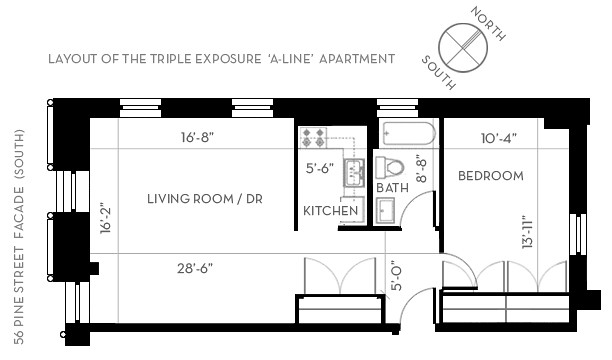This image is a detailed diagram of a rectangular apartment layout, presented on a white background with black imagery and text. The top of the diagram features the title "Layout of the Triple Exposure A-Line Apartment" in capitalized black text, spanning approximately two-thirds of the diagram's width.

On the left side of the diagram, aligned vertically, is the address noted in small black font: "56 Pine Street, facade (south)."

To the right of the title, there is a compass indicating directions with "N" roughly positioned at the two o'clock mark, and "S" at around seven o'clock.

The outer boundary of the apartment layout is depicted with thick black lines, representing the building's walls. Inside the rectangle, various rooms are labeled with their respective dimensions, all in the same black font used for the other text in the diagram.